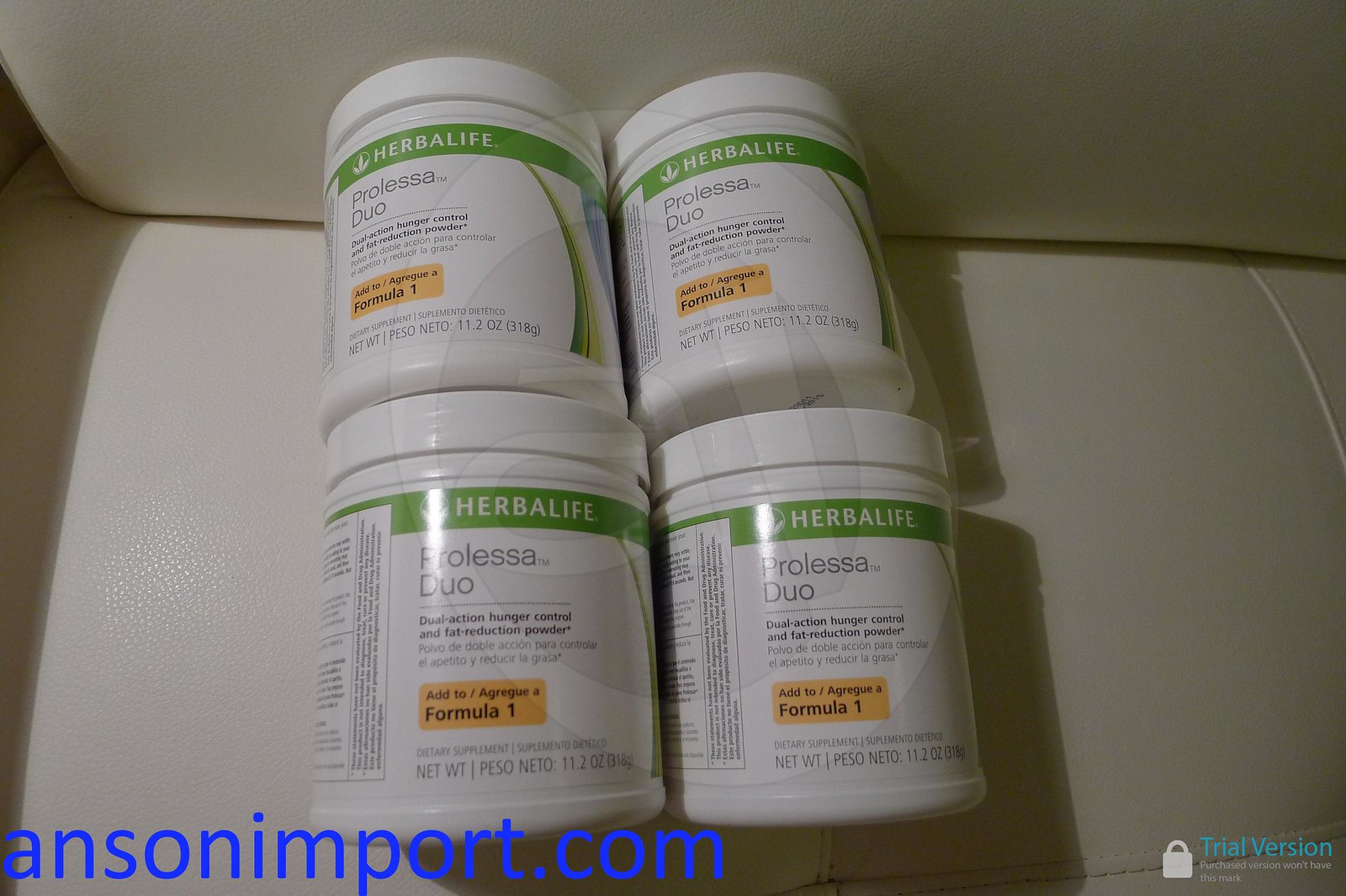The image showcases four identical white plastic canisters, each prominently branded with a green Herbalife logo at the top. The product is labeled "Prolessa Duo," a dual-action hunger control and fat reduction powder, with the text also presented in Spanish beneath. Each canister contains 11.2 ounces (318 grams) of the product and includes directions on the side, although they are partially obscured due to the angle and curvature of the containers. The canisters are arranged on a white leather surface, likely a couch or car seat. In the bottom left corner of the image, there is a watermark with the website "ansonimport.com," and in the bottom right corner, there is a blue label that reads "trial version" with a picture of a lock, indicating that the purchased version would not have this mark.